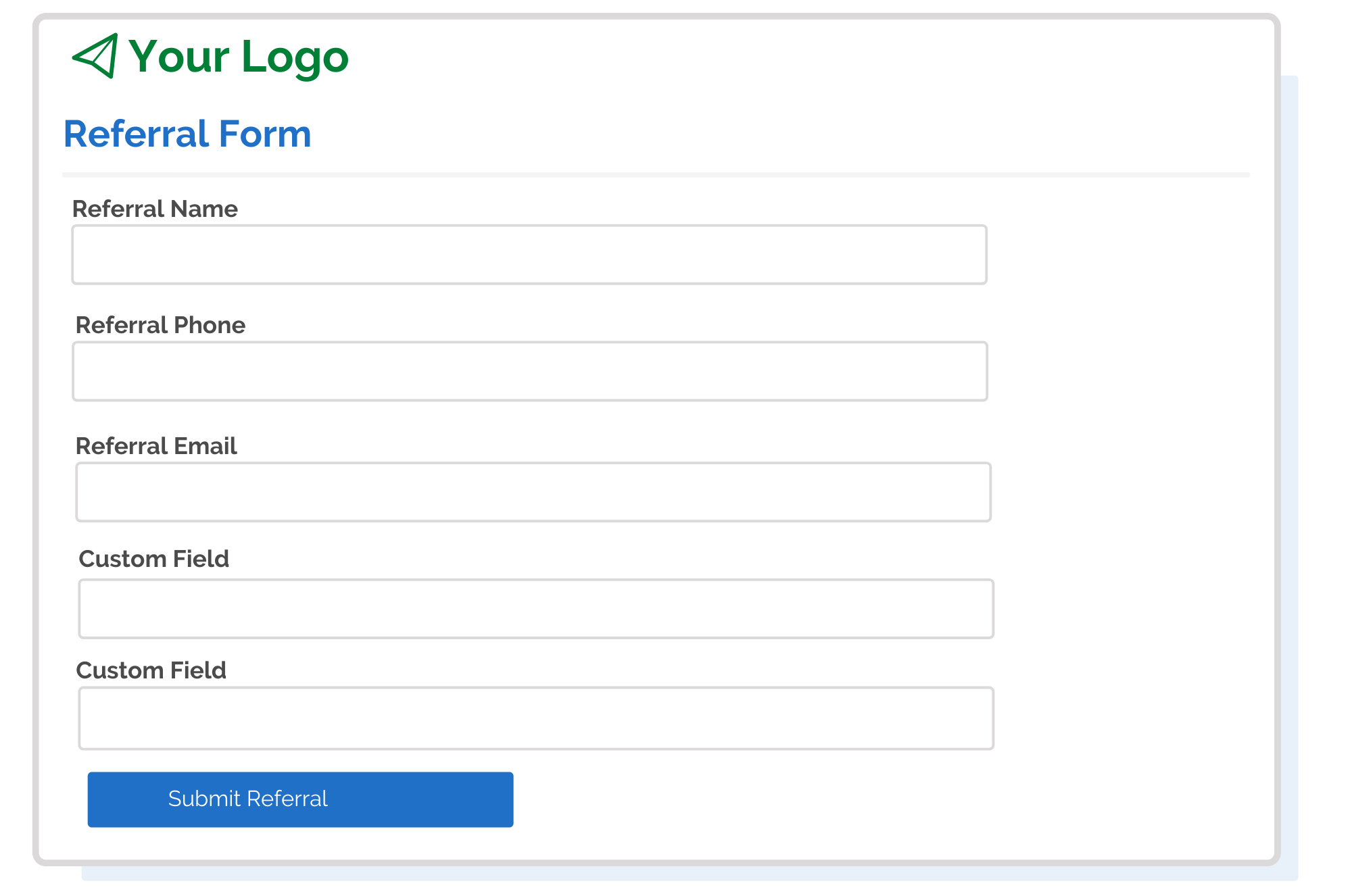This image depicts a referral form interface, presented as a rectangular white box with a subtle gray border. On the upper left corner, there is an icon of a paper airplane outlined in green, adjacent to the text "Your Logo" also in green. Below this, the title “Referral Form” is prominently displayed in blue, with a thin gray line separating this heading from the rest of the document.

The form contains several labeled fields:
1. "Referral Name" with an accompanying text box for inputting the name.
2. "Referral Phone" with a corresponding text box for entering the phone number.
3. "Referral Email" with a text box to type in the email address.
4. "Custom Field" followed by a text box for additional information.
5. A second "Custom Field" with another text box for further custom entries. 

All text boxes are currently empty. At the bottom of the form is a clickable blue button labeled "Submit Referral" in white text, designed to submit the completed form.